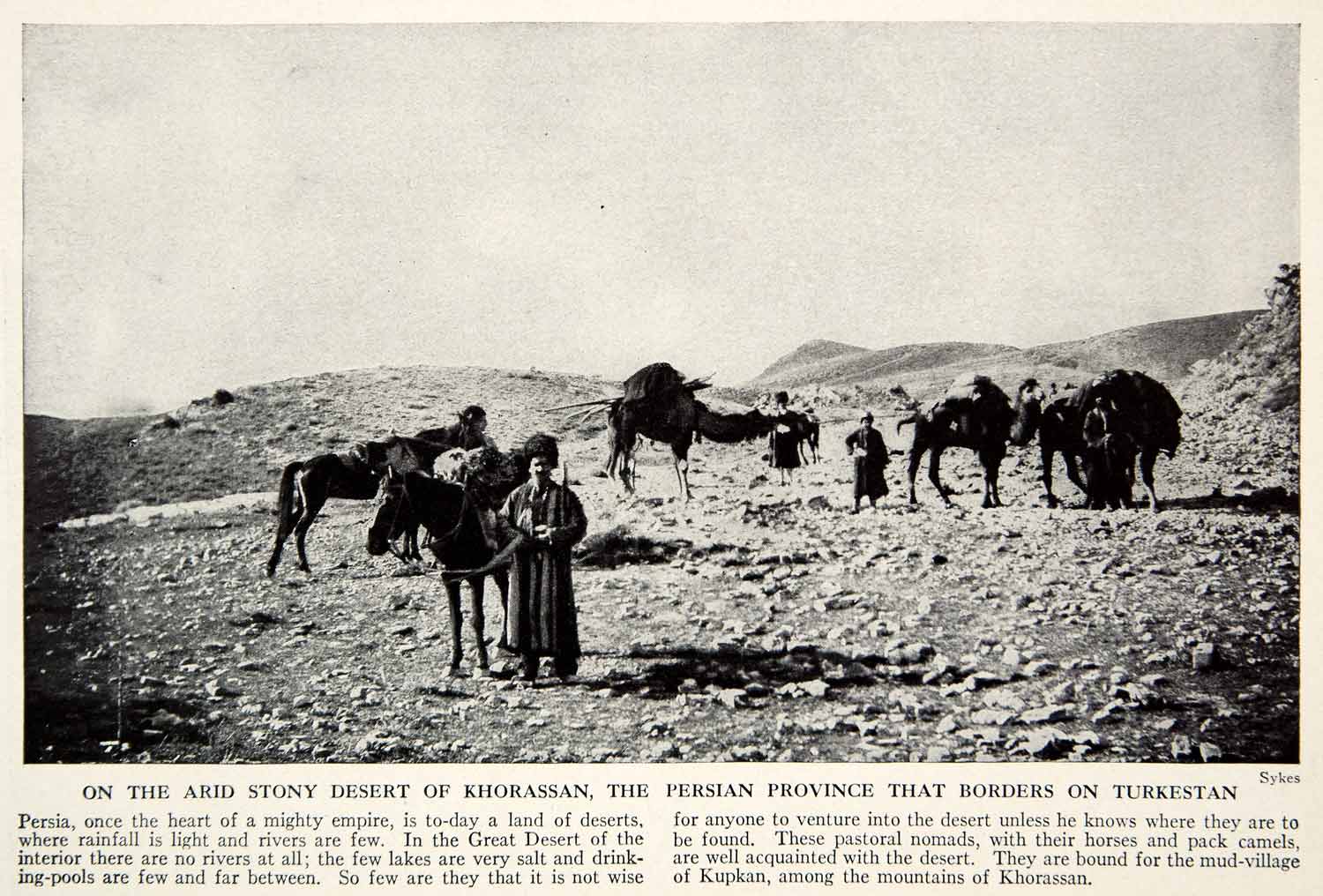This is a horizontal black-and-white photograph featured on a faded beige, old newspaper page. The image, which occupies most of the page, depicts a daytime scene in the arid stony desert of Khorasan, a Persian province bordering Turkestan. The landscape is barren with rocks scattered on the ground. There are five or six men dressed in robes and turbans, standing alongside several camels and horses, all of whom appear to be looking at the camera. Intriguingly, the camels are loaded with various items, indicating travel or trade. The newspaper text beneath the image provides a detailed context, stating, "On the arid stony desert of Khorasan, the Persian province that borders on Turkestan." It elaborates further, explaining the harsh environment of Persia, once a mighty empire, now a land of deserts with little rainfall and scarce water sources. These pastoral nomads with their horses and camels are familiar with the desert and are journeying to the mud village of Kubkhan in the mountains of Khorasan. The word "Sykes" is also noted beneath the photograph.